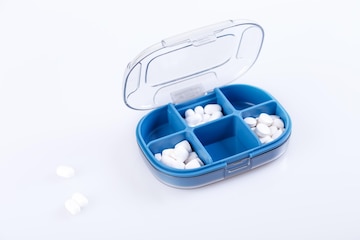The image depicts a blue, oval-shaped pill container with a transparent, open lid displaying patterns. The interior of the container is divided into six compartments, each designed as either square or square-like with rounded corners. Three of these compartments, specifically the bottom right corner, upper middle section, and bottom left corner, are filled with equal amounts of white pills or mints. Additionally, three identical white pills or mints are scattered to the left of the container. The base of the container appears to be clear plastic beneath the blue divisions, and the lid seems to be designed to snap shut securely.